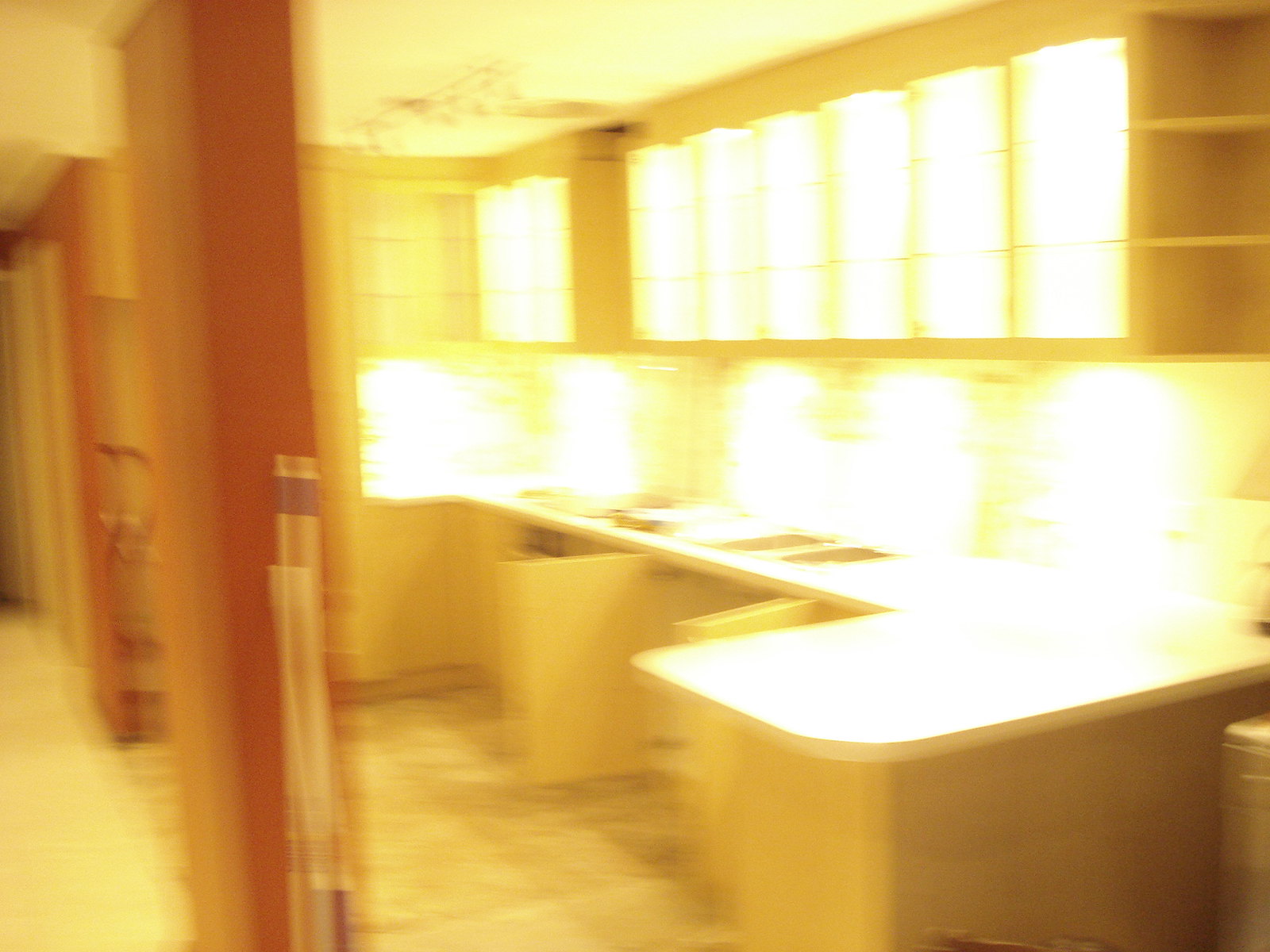The image displays a kitchen counter that appears to be blurred. The brightly lit space is illuminated from below a row of cabinets above the sink, as well as from inside overhead glass storage cabinets. The kitchen features open shelving on one side and the counter forms a wide U-shape. There are two sinks visible on the counter, and beyond them, potential stove fixtures, though they are indistinct due to the blurriness. The kitchen counters are white, and the room is bathed in a yellowish hue. The floor behind the sink seems to be tiled, and two brown wall partitions frame this open kitchen area. On one side, a walkway with white or beige flooring, possibly a rug, provides access to the kitchen space.